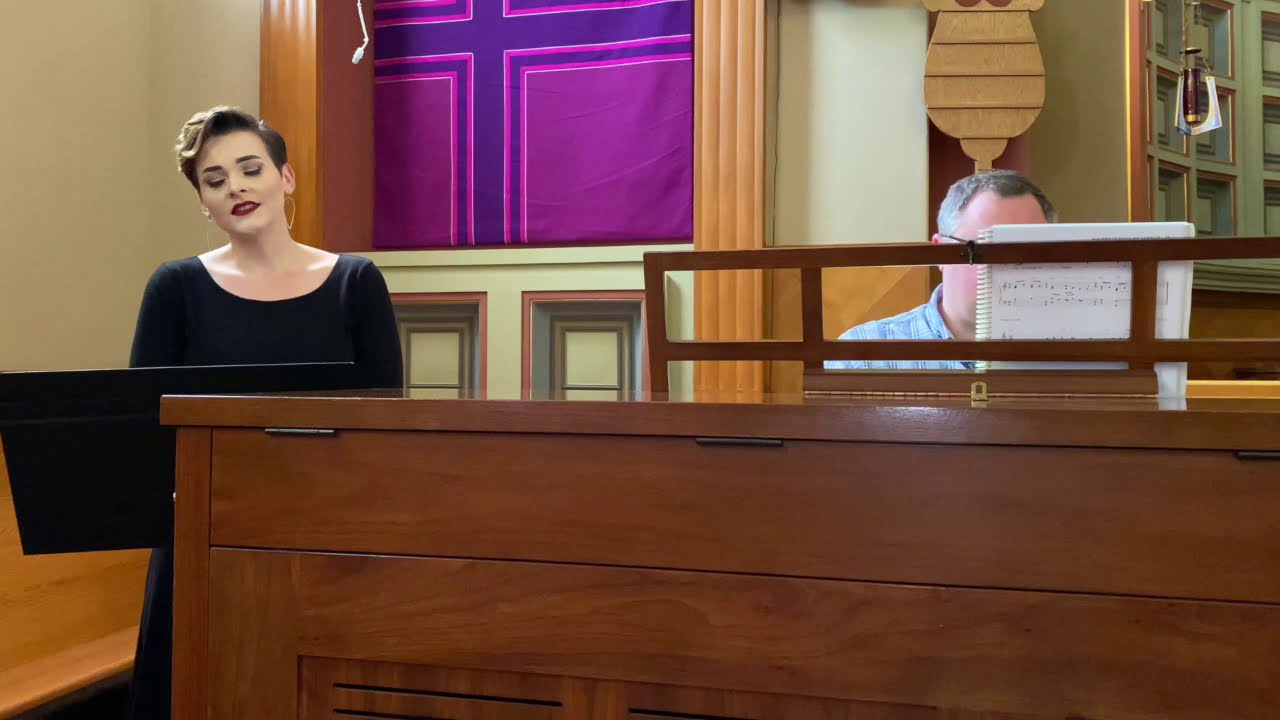In the image, there is a detailed scene of two musicians inside what appears to be a church setting. To the left, a young Caucasian woman with short brown hair, red lips, and big hoop earrings is standing behind a black music stand, likely singing or beginning to sing, as her mouth is slightly open. She is dressed in a black dress and positioned in front of a reddish wood podium. Behind her, a man with short gray hair, glasses, and a blue shirt is seated on a bench, playing a large brown piano. His face is obscured by a white music notebook placed on the piano's top. The church's tan and brownish walls feature a purple cross banner, and touches of pink and blue decorations are visible in the background. The overall setting, including wooden pedestals and the detailed backdrop, signifies a classic and serene atmosphere conducive to musical performance.